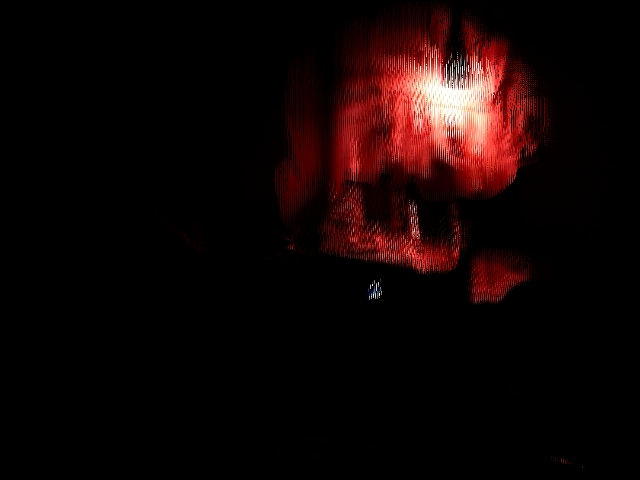The image predominantly features a dark, almost black background. Near the top right section, vivid shapes in varying shades of red stand out against the darkness, creating a striking contrast. The reds range from deep, darker hues to lighter, more vibrant tones. At the center of this reddish area, an intense brightness emerges, showcasing light yellows and whites that suggest a source of illumination behind or within the shapes, making them glow. A smaller, distinct red shape is positioned slightly apart from the larger mass, adding a sense of depth and separation. Additionally, a curious, small, white shape resembling a 'Z' is visible amidst the composition, providing a unique focal point that diverges from the surrounding reds. The overall composition gives the impression of a mysterious, illuminated form emerging from the shadows.